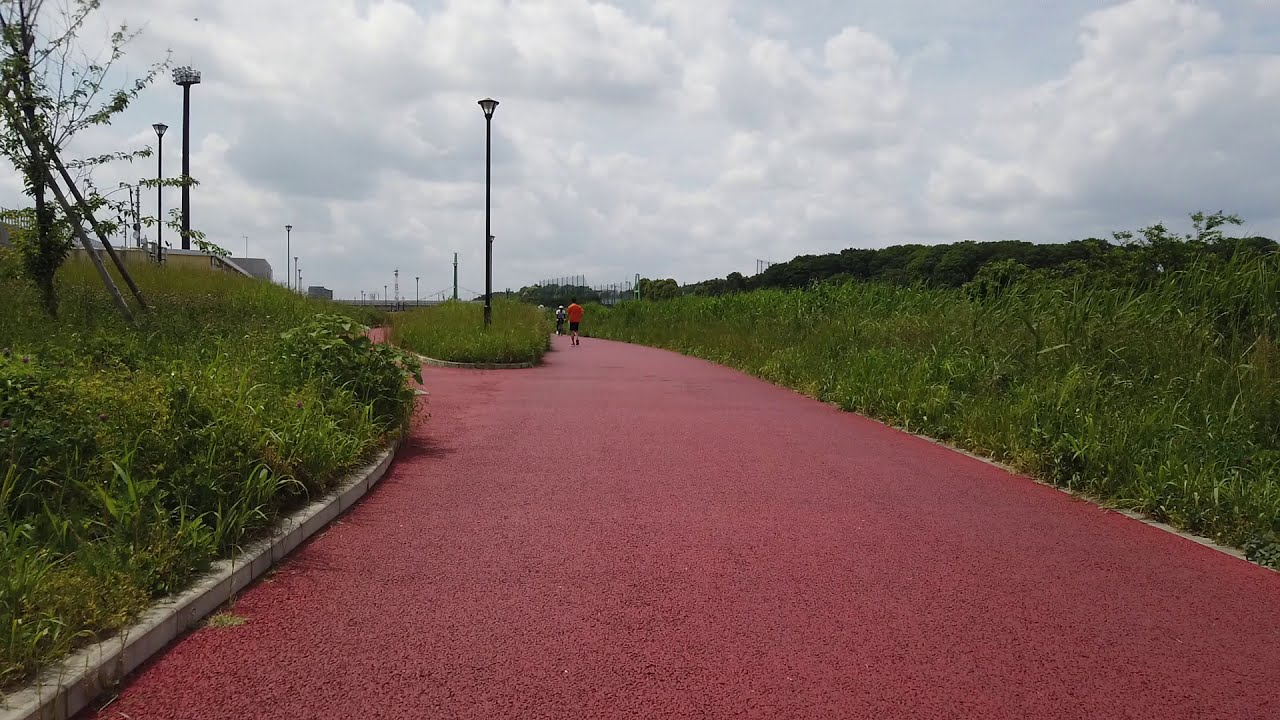The photograph is a vibrant and detailed depiction of a scenic outdoor pathway, colored a striking rich maroon and made from what appears to be a crushed tire surface. This pathway curves its way through the center of the image, starting wide in the foreground and narrowing as it recedes into the distance. The path is of ample width, suggesting it is designed for pedestrians rather than vehicles. On either side of the pathway, a white curb lines the edges, beyond which lies an abundance of lush greenery, including various shrubs, trees, and other plantings. 

Notably, there is a green island slightly to the left of the center, adorned with a black lamppost, and more lampposts can be seen stretching into the background. In this central area, a tree supported by sticks indicates ongoing landscaping efforts. To further enhance the natural beauty, the backdrop features mountains blanketed with trees, adding depth to the scene. 

There are a few people visible, primarily to the right of the green island, who seem to be jogging or walking along the pathway, suggesting this is a popular area for outdoor activities. The sky overhead is softly lit, a blend of light blue hues intermingled with thick, fluffy white and gray clouds, bringing a serene ambiance to the entire scene. The rich palette of colors includes shades of black, white, gray, blue, green, yellow, red, orange, cranberry, and maroon, making the image vivid and visually appealing. Photographic in style, this color photograph captures a moment of realism and tranquility during daytime, effectively inviting viewers into its lush, serene environment.